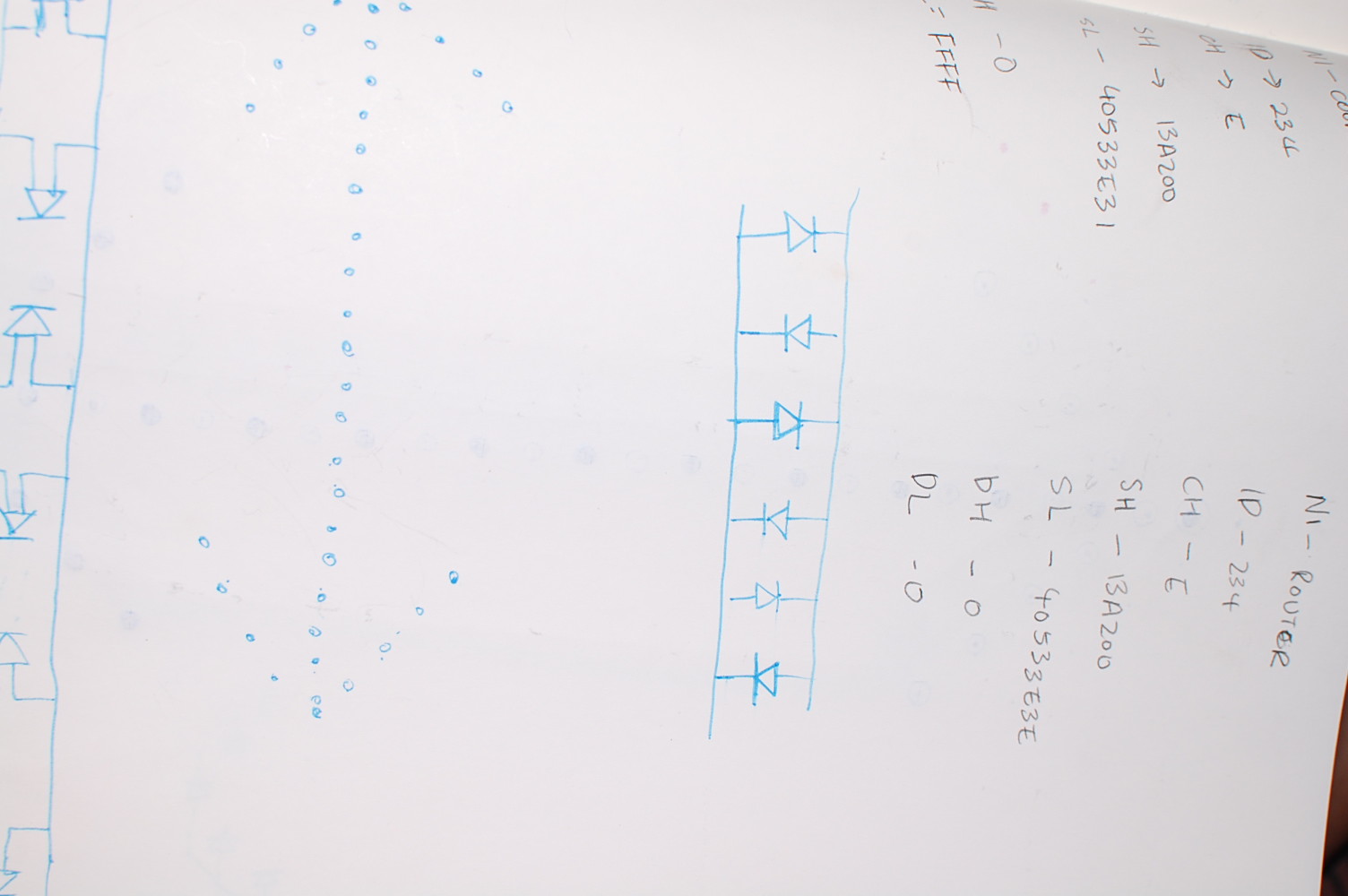The image features a rectangular photograph of a notebook page filled with handwritten notes, taking up a significant portion of the frame. The photograph has a landscape orientation, with the top and bottom sides measuring twice the length of the left and right sides. The central subject of the image is a white, slightly curved page from a notebook, captured at an angle. The curvature hints at the page being part of a bound notebook, with a glimpse of the adjacent page visible in the top right corner.

The notebook page is tilted such that the top of the page points towards the right, while the bottom points towards the left. The handwritten notes, inscribed in pencil, are predominantly located on the right side of the page. Due to the angled perspective, the text appears sideways. The visible and clearly readable text consists of a sequence of alphanumeric codes and designations, specifically: "NI-ID-234-CH-E-SH-13A20D-SL-40533E31-H-0 FFF NI-ROUTER-ID-234-CH-E-SH-13A200-SL-40533E30-DH-0-DL-0."